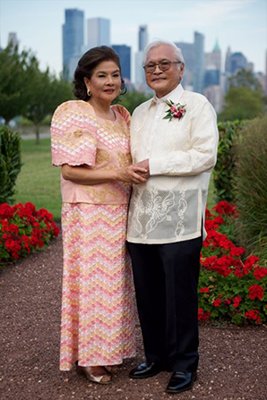In the image, an older Asian couple in their 50s stands hand-in-hand on a rock pathway lined with red roses and manicured bushes. Both dressed elegantly, the man on the right wears a white button-up shirt with a flower bouquet pinned to the pocket, black dress pants, and black dress shoes. He has gray hair, glasses, and is slightly turned toward the woman. The woman on the left, with short dark hair, wears a peach and pink striped zigzag dress with prominent shoulder pads and a long skirt, accessorized with fancy shoes and earrings. She is also slightly turned toward the man. The background showcases a vibrant cityscape of skyscrapers under a blue sky with sparse white clouds, framed by green trees. The scene is both intimate and picturesque, with the main focus on the affectionately posed couple.